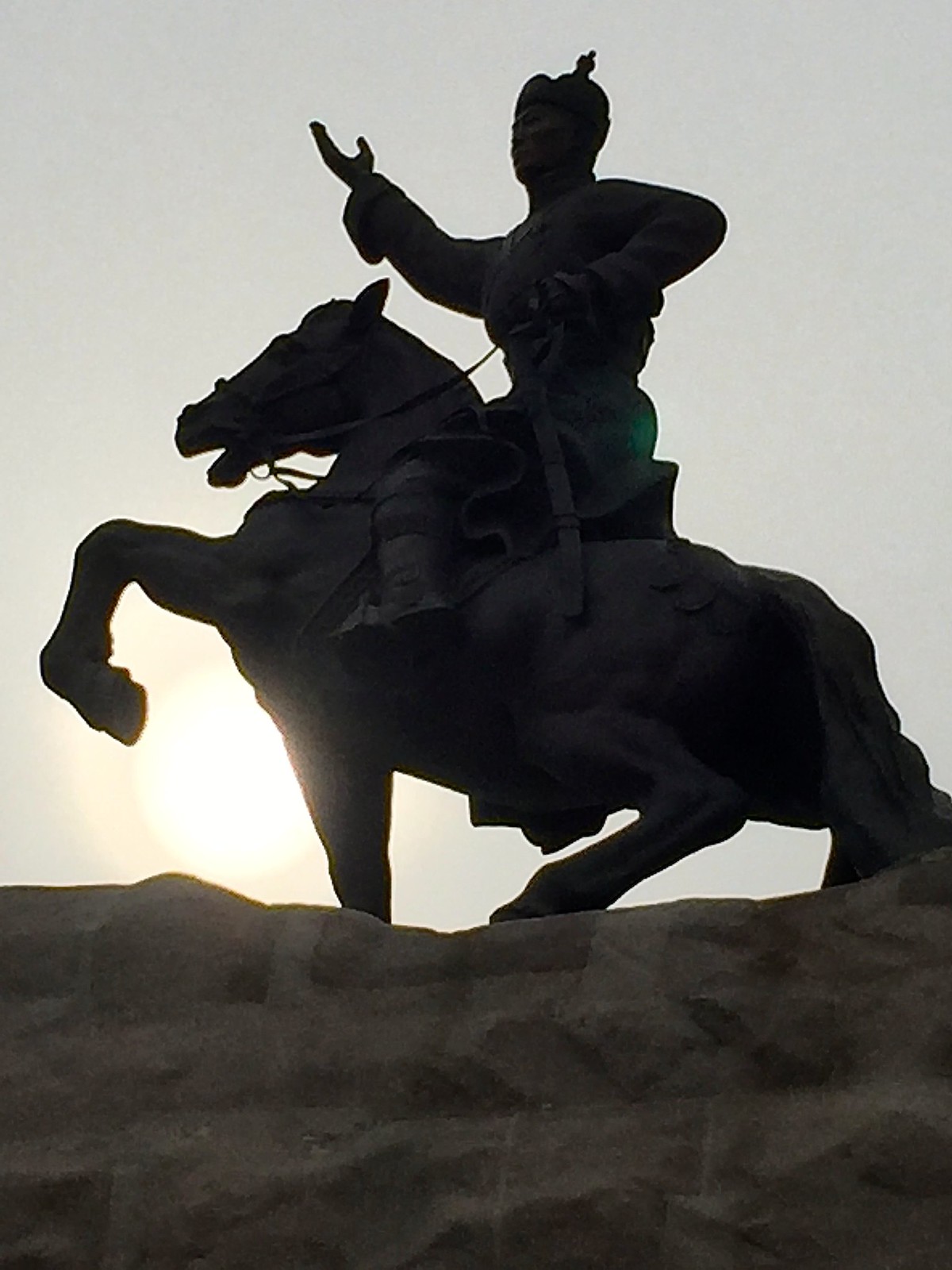The photograph captures a striking outdoor statue of an Asian warrior, possibly Chinese or Tibetan, mounted on a powerful horse. Viewed from a low angle, the silhouette is set against a gray, sunlit sky, emphasizing the striking features of the statue. The warrior, adorned in long pants and what appears to be skirt-like attire, is depicted with a distinctive, tall helmet featuring a pointed crown. His face remains obscured in shadow. Mounted on a heavy saddle, the warrior grips the horse's bridle with his left hand, while his right arm extends upward at shoulder height, his hand pointing towards the sky. His head is slightly tilted to the right, aligning with his raised hand, as if indicating a direction or issuing a command.

The horse is sculpted magnificently, with an arched neck and a large head, its mouth open as if in mid-whinny. The right foreleg of the horse is dramatically raised and bent, adding to the dynamic posture of imminent motion, while its left foreleg holds steady on the ground. The hind legs appear bent, suggesting that the horse might be ready to rear up. The stone pedestal on which the statue stands is jagged and craggy, contrasting with the smooth silhouette above. A bright strobe of sunlight penetrates the scene just beneath the raised foreleg of the horse, creating a dramatic illumination that enhances the overall majestic and commanding presence of the statue.